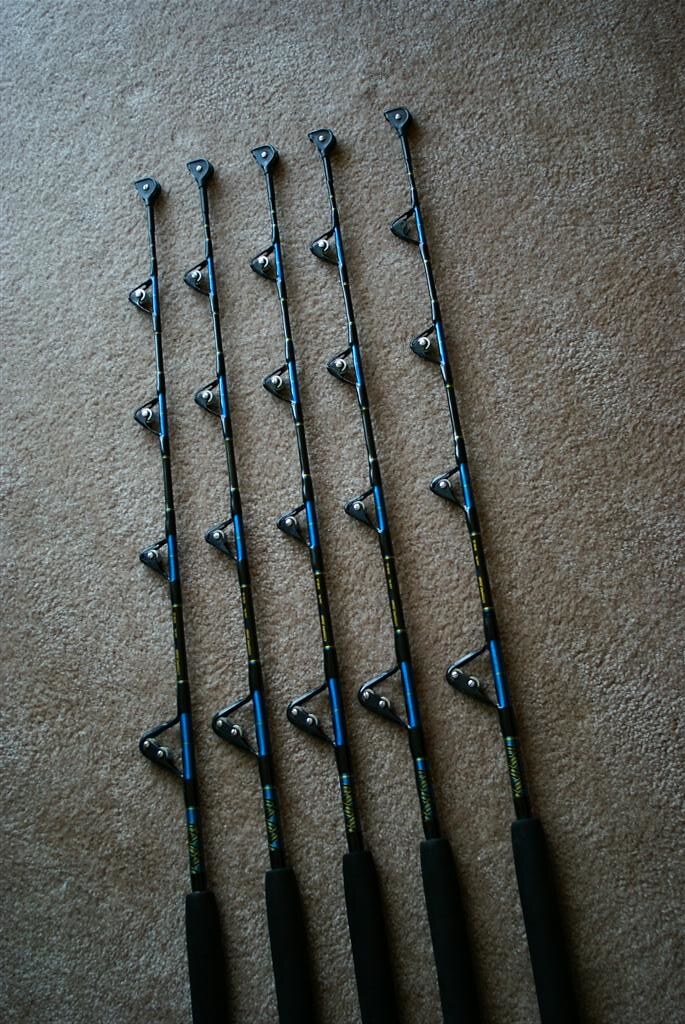The image is a realistic photograph of a vertical rectangular shape, featuring a beige carpet that appears lighter towards the top left and darker towards the bottom right, likely due to lighting and shadow. Arranged parallel to one another, there are five identical long, thin pole-like objects spanning almost the entire height of the image. Each object has a thicker handle, perhaps foam-coated, at the bottom right.

The rods are primarily black with blue trim and have distinctive features along their length. Starting from the bottom near the handle, there are four evenly spaced triangles along each rod. Each triangle contains small ball bearings or circular metallic objects. Specifically, the bottom triangle has two ball bearings, while each of the next three triangles contains one ball bearing.

At the tip of each rod, there is a small circular or oval shape featuring a yellow dot in the center. The poles also seem to have some illegible writing on them. The repetitive and symmetrical arrangement of these items, combined with the detailed appearance of their components, adds an intriguing and somewhat mysterious element to the scene.